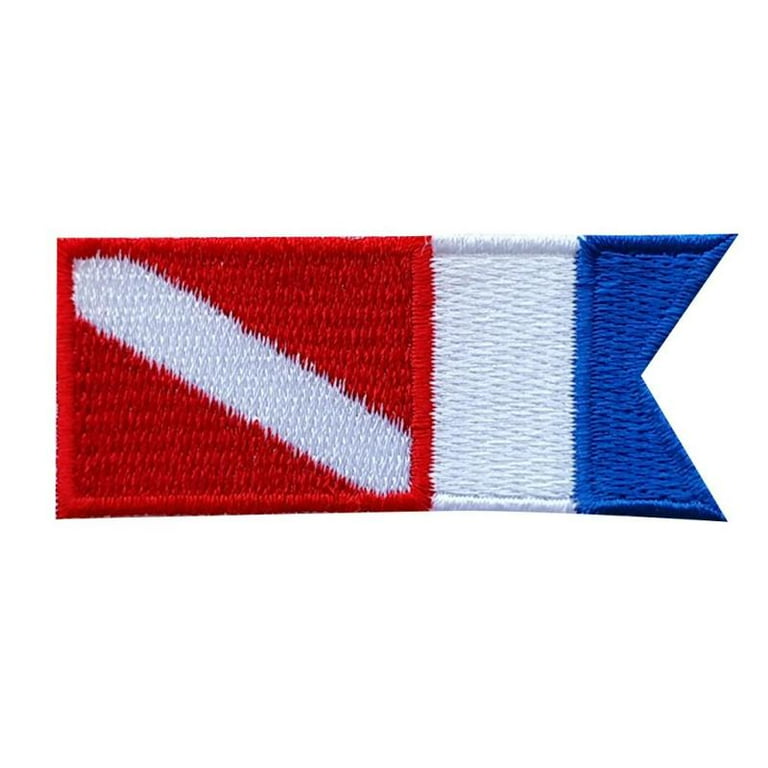The image features a vibrant embroidered or iron-on patch designed for clothing, such as jackets or jeans. This distinctive patch, set against a white background, draws immediate attention to its unique red, white, and blue color scheme. On the left side, a significant red rectangle, three times the size of the other sections, dominates the design. This red section is intersected diagonally by a white stripe running from the top left to the bottom right corner. Adjacent to the red rectangle is a smaller, solid white rectangular section. The rightmost part of the patch is a blue area, intricately shaped to resemble an inverted triangle or the letter "K," adding a touch of geometric complexity. The overall shape of the patch is nearly rectangular, with the notable blue section creating a unique form. This patch, possibly symbolic of a flag, stands out with its vivid colors and textured, fuzzy material.